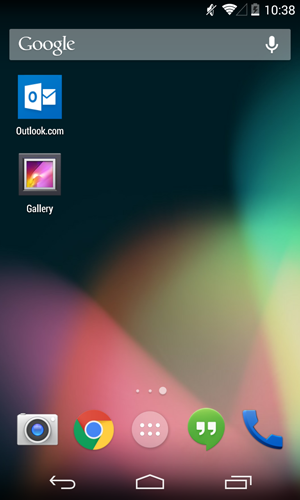The image depicts the home screen of an Android smartphone set against a blackish background with highlighted accents of green, red, and orange. Prominently placed at the top is the familiar Google search bar, affirming its Android OS. Several well-known app icons populate the screen. Among them is the Outlook.com icon, distinguishable by its traditional envelope symbol on a blue square. There's also a Gallery icon symbolized by a picture frame with hues of purple and orange inside it.

At the bottom of the screen, a row of essential app icons is visible. These include a Camera, the Google Chrome browser marked by its signature red, green, yellow, and blue circular design, and a green messaging app icon represented by a speech bubble with two apostrophes. Additionally, there's an old-fashioned blue telephone icon for making calls. The central icon in this app row seems to be for switching tabs or displaying the phone's recent apps menu.

Further below, the device's navigation bar includes a central home button, a back left arrow on the left, and a square overlapping another square on the right, possibly for multitasking.

The time displayed on the device is 10:38. The battery icon indicates low power with a lightning bolt symbol, suggesting it's charging. The phone is connected to a Wi-Fi network with full signal strength, and it's in silent mode as indicated by the muted speaker icon.